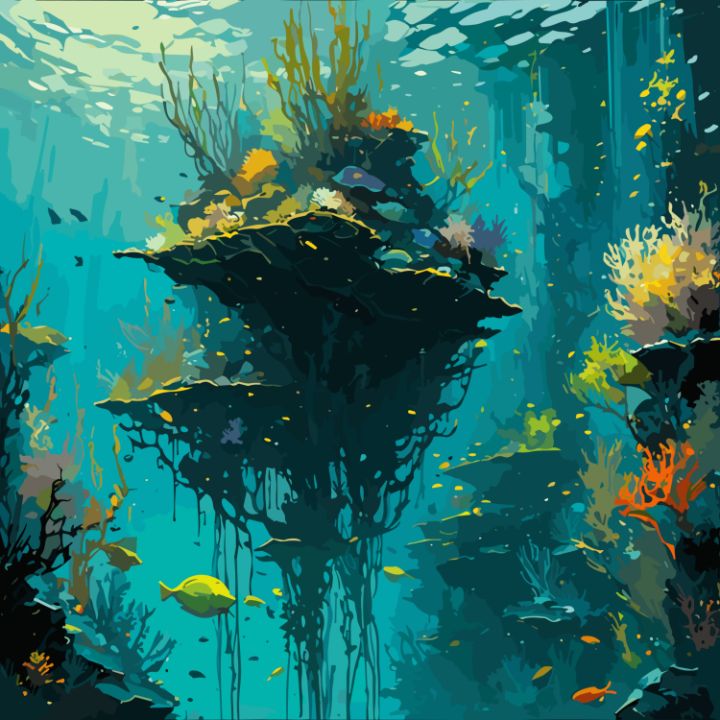This artwork depicts a vibrant underwater scene brimming with an array of colors and marine life. The scene is set under the sea, enveloped in hues of blue and green. The upper section features lighter yellowish-green areas that blend into a predominantly light green expanse, with variations hinting at a greenish-blue. On the right side, shelves of coral or plants, in bright oranges and yellows, cascade downward like steps. There are also rock shelves interspersed with colorful coral, showcasing oranges, yellows, and touches of green. 

At the center of the composition, a floating island of rock emerges, adorned with gray roots that dangle beneath it. The underside of this rock is black, but it's contrasted by green plants and accentuated by splashes of yellow and blue colors. Sprinkled throughout the scene are fish in dynamic shades of blue, orange, and yellow, adding motion and life. In the lower left part of the image, there are hints of brown coral, offering more earthy tones amid the vibrant marine ecosystem. The entire scene paints a vivid, almost watercolor-like portrayal of the underwater world, rich in color and teeming with aquatic flora and fauna.